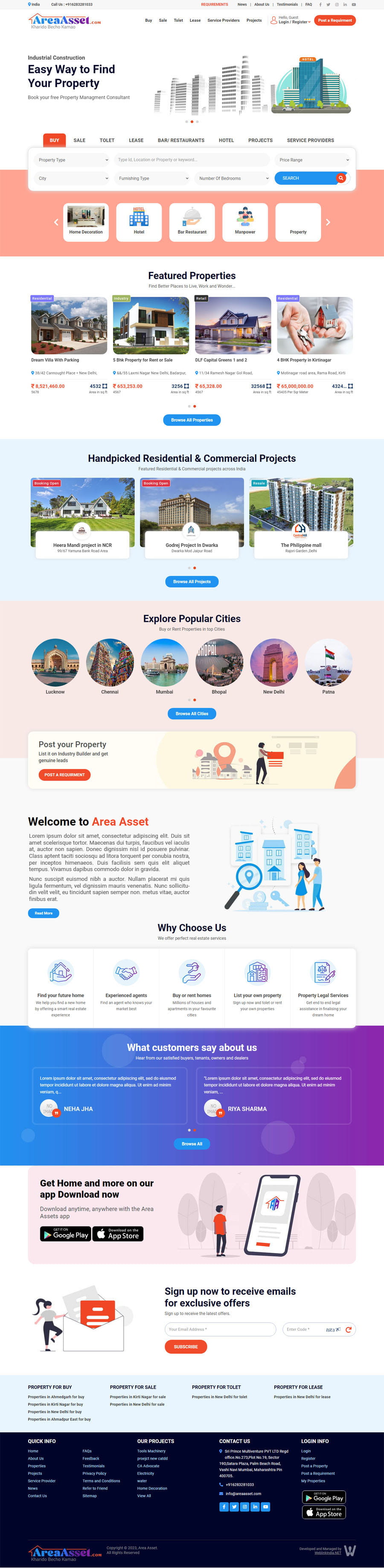The image features a primarily white background. At the top-left corner, there is a box with blue and purple print, displaying an image of a large building. Adjacent to this, there's another image of a blue-colored building surrounded by greenery. Below that, a small red box with white print is visible.

Further down, there is a light blue box containing a button at the bottom, which is blue with a red end. Near this, a pink box features five selectable options and some icons, accompanied by a picture. Below the pink box, a white box showcases four colored images, with the last one displaying a hand holding an object, and some print below it. 

A blue box follows, containing three images of large buildings with white captions under each. At the bottom of this blue box, there is a blue button. Moving on, another pink box with six images invites viewers to explore popular cities, accompanied by a blue button underneath. There's also a white box with a red button, featuring two small pictures and a semi-circle on the side. 

Furthermore, there's a section labeled "Welcome" that resembles artwork, with a magnifying glass and two blue figures. Another white box contains five small icons. Below this, a bright blue box features two buttons and another blue button at the bottom. Toward the end, a purple box contains two black buttons, an image of a person, and a tall telephone. Additionally, there's an image that resembles an envelope with a red item inside and a red button.

Finally, a light blue strip features black elements and five small blue buttons at the bottom.